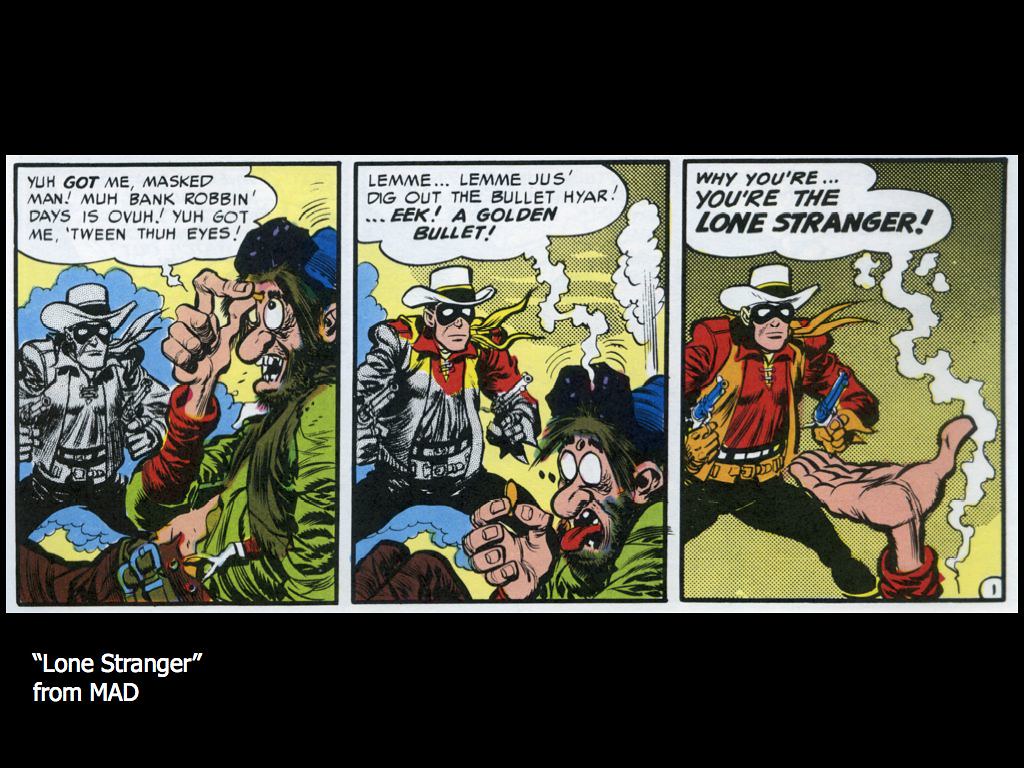This is a detailed three-panel comic strip titled "Lone Stranger" from MAD magazine. The first panel features two illustrated characters: a cowboy in a costume, enveloped in a blue and gray cloud of smoke, and a disheveled man with a large rounded nose. The man with the scruffy appearance, who looks like a sheriff, exclaims in a panic, "You got me, masked man. My bank robbing days are over. You got me between the eyes." The second panel zooms in on the disheveled man, now at the bottom of the frame and appearing even more panicked. He frantically says, "Let me just dig out the bullet here... Eek, a golden bullet!" while holding the gold bullet in his fingers. His eyes are wide and white, his mouth open with his tongue out in shock. The cowboy on the left is more visible, with smoke covering the bottom half of his body in a black-and-white shading. The final panel shows the cowboy, still taking the same pose with his pistols held confidently in each hand. The disheveled man's hand, appearing just in the bottom right corner, still clutches the bullet. He declares in astonishment, "Why, you're the lone stranger!" The speech bubble is prominent, while the text at the bottom left of the image states, "Lone Stranger from MAD."